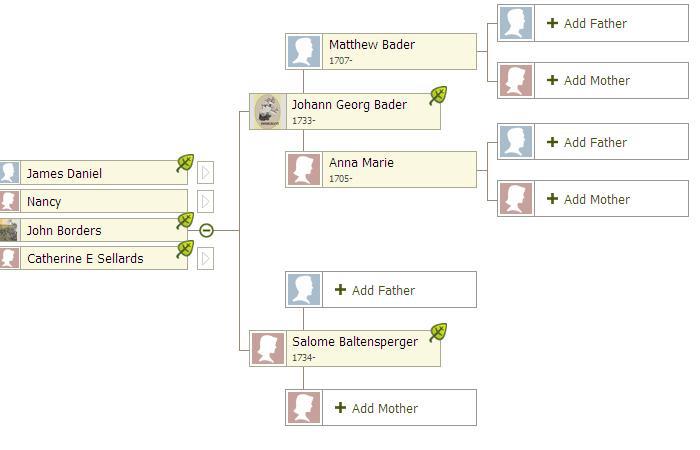This color image is a detailed genealogy chart, likely from Ancestry.com. On the far left, four names are listed: James Daniel, Nancy, John Borders, and Catherine E. Sellards, each accompanied by a leaf symbol. The chart focuses on the lineage of John Borders, whose name is highlighted. John Borders' father is Johann George Bader, born in 1733, and his mother is Salome Baltensperger, born in 1734. Johann George Bader’s parents are Matthew Bader, born in 1707, and Anna Marie, born in 1705, both of whom have no further listed ancestors. Salome Baltensperger does not have any listed parents. Leaves next to several names, including Catherine E. Sellards, John Borders, Johann George Bader, and Salome Baltensperger, indicate probable connections to Ancestry.com’s database.